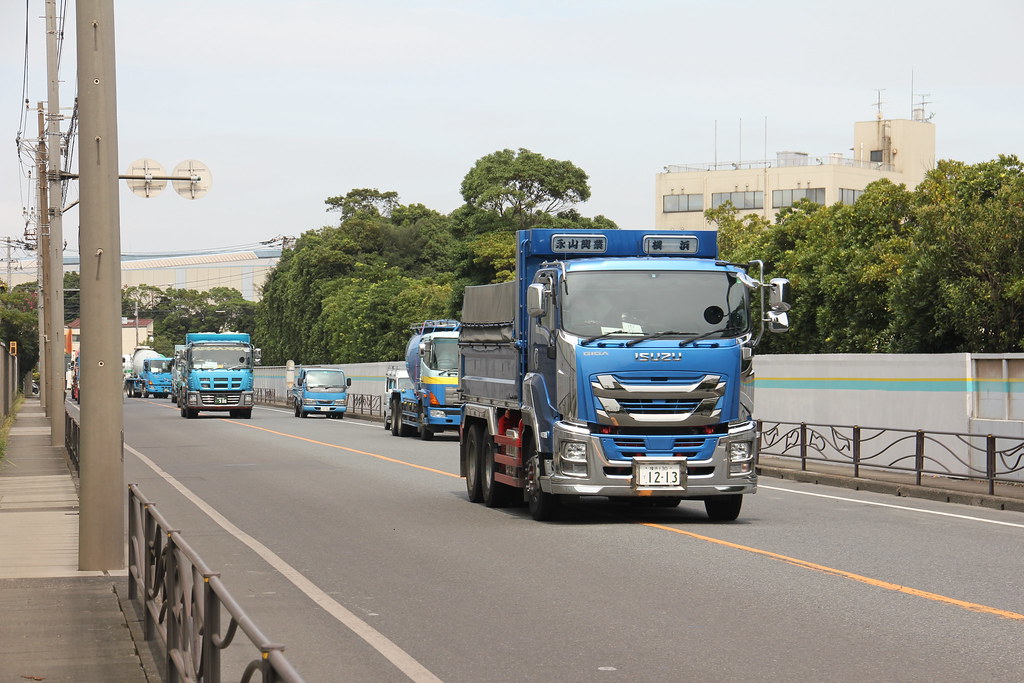This is a detailed photograph of a highway scene, likely set in a European city, showing a procession of large, blue industrial trucks driving towards the camera. The highway is paved in typical light gray asphalt with a solid yellow line running down the center, indicating a one-way route. On the left side of the road, there are telephone poles and a grayish sidewalk, while the right side features leafy green trees and metal railings, as well as a low, patterned fence.

The truck closest to the foreground is a dark blue Isuzu dump truck with chrome detailing and some Oriental writing across the top. Behind it, a sequence of blue vehicles follows: a lighter blue truck, possibly another dump truck; a blue pickup truck; a turquoise truck; what seems to be a van; and a light blue cement mixer.

In the backdrop, a large, industrial-looking building looms, partially hidden by trees. A few small personal vehicles are parked on the right side of the road near the railing. The scene includes a beach with a boat visible on the sand, adding an interesting mix of urban and serene elements to the image. The overall atmosphere portrays a busy highway with various types of industrial vehicles primarily in the shades of blue, moving towards the viewer.